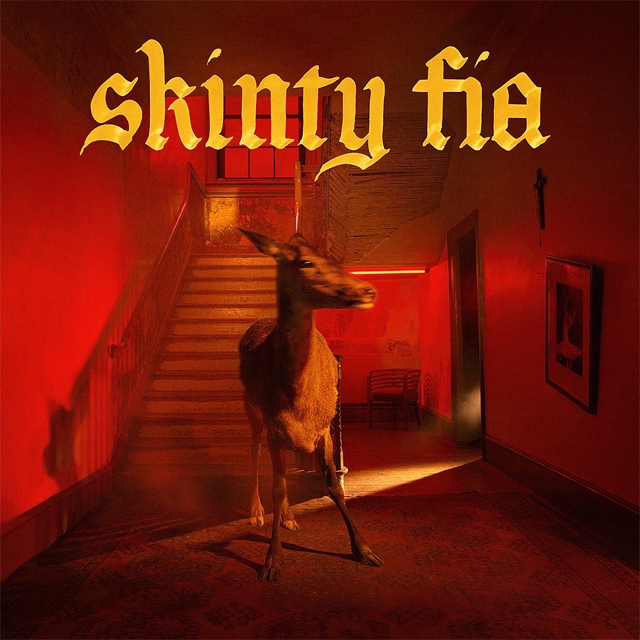The image appears to be a square, likely cropped from a website, and resembles a record or CD cover. It prominently features a blurry deer standing on a piece of carpet at the foot of a wooden stairway in a downstairs room. The entire room is bathed in eerie red lighting, possibly from a red light source, casting a shadowy and unsettling atmosphere. The word "Skinty Fia" is written in calligraphic yellow letters across the top of the image. On the right side of the deer, there's a doorway with a beam of light shining through, a cross hanging on the wall, and a picture beneath it. A chair is positioned in the corner of the room. The stairs leading up are wooden and appear decrepit, with the first floor also featuring wood and ornate wooden molding. A fluorescent light is visible behind the deer, adding to the odd and creepy ambiance of the scene.